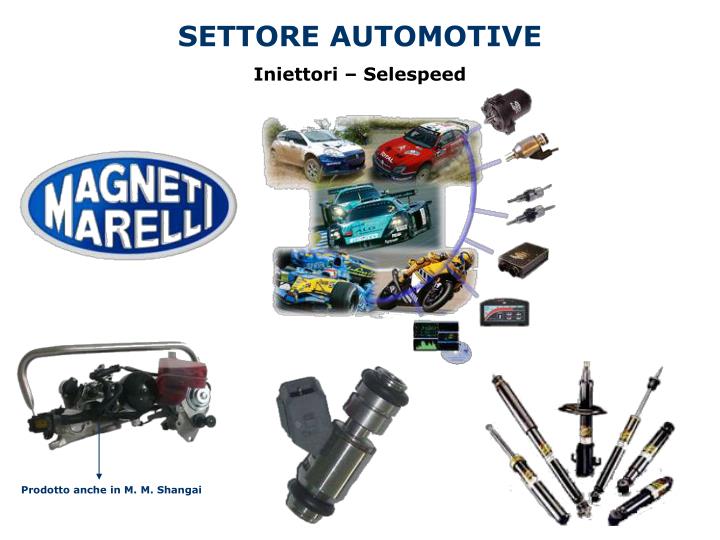This advertisement for C-Tour Automotive prominently features the name "Inietori-Celespeed" in black letters below the main title. The central image showcases a vibrant collage of high-speed race cars and motorcycles, evoking a sense of speed and performance. Along the right-hand margin of the image, various automotive parts are arranged, adding a technical and mechanical aspect to the ad. To the left, a blue oval shape features "Magneti Marelli" in white letters. Below the main image, three detailed pictures of auto parts are displayed: the left one is unidentified, the middle one appears as a silver cylinder, and the right one is a black and gold cylinder-shaped part with additional objects extending from it, resembling automotive components. The advertisement is filled with an assortment of images and labels, enhancing its appeal to automotive enthusiasts.